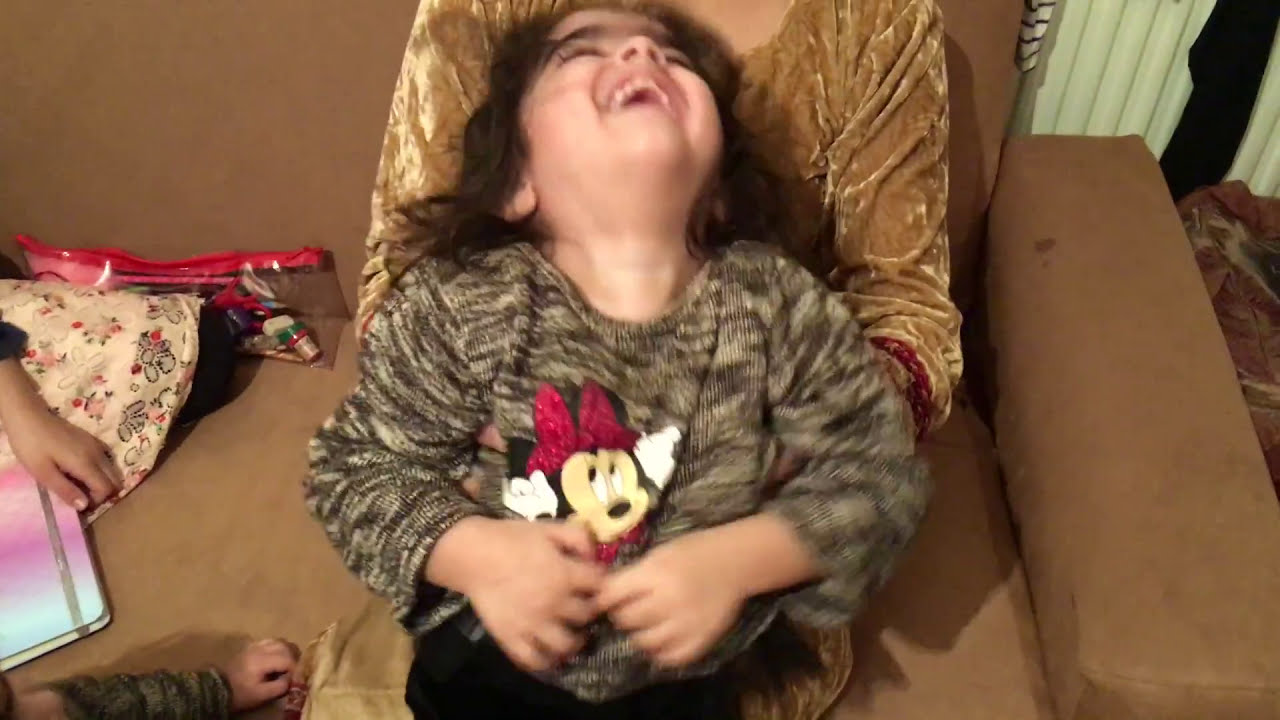A young girl with long black hair, around three to five years old, sits on an older person’s lap, who is likely her mother or grandmother. The child's face is tilted back, and she is laughing joyously. She wears a gray and black sweater adorned with a Minnie Mouse design, featuring a pink bow. The two are seated on a plush brown suede or velvet-style couch. The older person, whose face is obscured, wears a gold shirt. In the bottom left corner of the image, another child's left arm and hand rest on the couch. Beside this child’s hand is a right hand holding a pink, purple, and blue binder placed on the couch. Also on the couch is a translucent bag with a red zipper, which appears to contain makeup. In the background, green curtains are faintly visible on the right side of the image. The joyful energy of the scene is amplified by the motion blur on the girl's hands and face, capturing a moment of pure happiness.